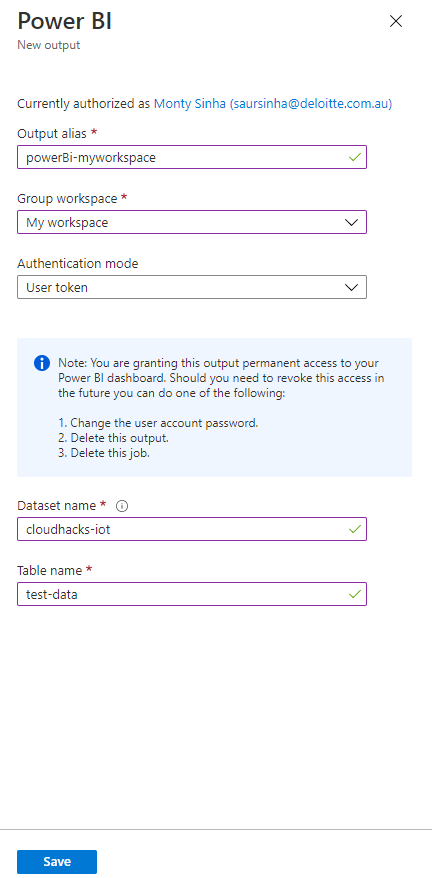"Image Description: The image displays a detailed interface of a software application featuring an authorization page.

At the top left corner, in simple black text, it reads 'Power BI'. Directly below, it says 'New Output' followed by 'Fully authorized as Monty Sinha (saur.sinha@deloitte.com.au)'.

Below the authorization details, there's a label for 'Output Alias' marked with a red asterisk indicating a required field. It reads 'Powered by My Workspace' with a checkmark at the end for confirmation. Next, another label titled 'Group Workspace', also highlighted with a red asterisk, states 'My Workspace'.

Further down, the 'Authentication Mode' is specified as 'User Token'. Towards the bottom, two additional input fields are displayed: 'Dataset Name', marked with a red asterisk, reads 'CloudHacks IoT', and 'Table Name' indicates 'TestData'.

Prominently, a large blue box communicates an important note: 'You are granting this output permanent access and other associated permissions.'"